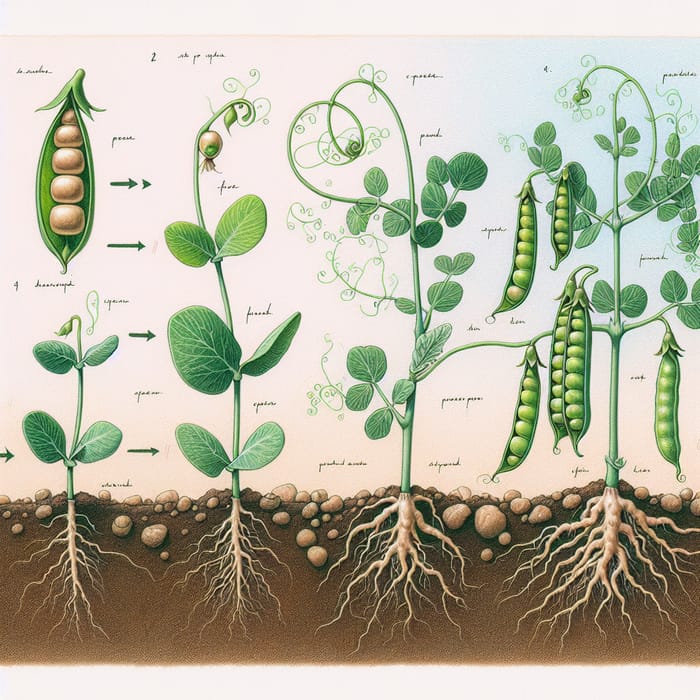This artist's illustration, balancing between realistic and cartoony, vividly depicts the growth stages of a pea plant. In the top left corner, a golden-hued open pea pod reveals peas lined up in a row. The main focus is on four stages of the plant's development, shown from left to right. The first stage presents a young, immature plant with a few leaves and a budding root system. Moving right, the second stage captures a slightly taller, juvenile plant, sporting two sets of leaves. The third stage introduces viney tendrils emerging from the top, indicating further growth. The final stage illustrates a mature pea plant, boasting multiple pods and a robust root system underground. The vibrant, infographic-like drawing offers an educational and visually engaging overview of the pea plant’s lifecycle.